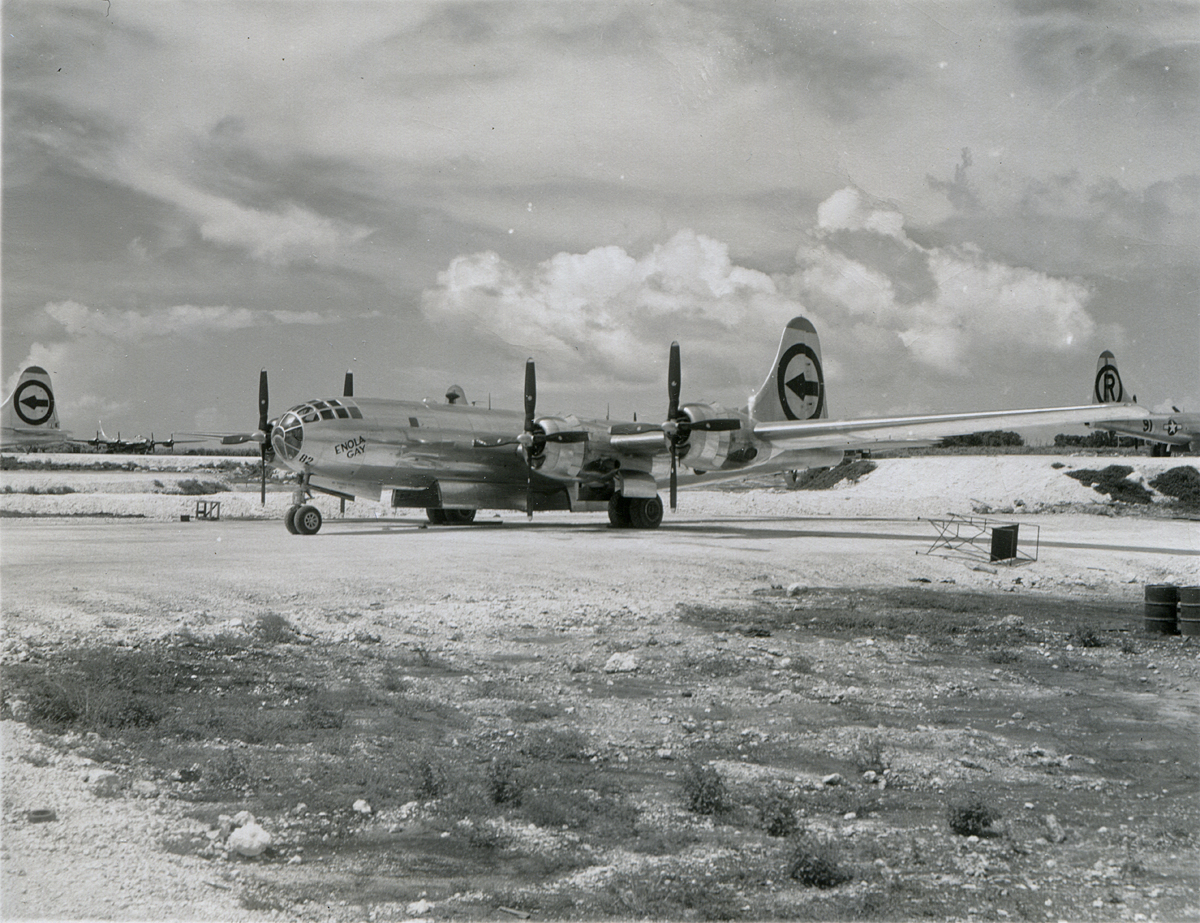This black-and-white photograph captures a striking image of the Enola Gay, the renowned four-propeller aircraft that dropped the atomic bomb on Hiroshima. The bright, chrome-finished plane is prominently featured in the center of the image, facing left, with its name "Enola Gay" clearly visible by the cockpit. Situated on a flat, gravel-strewn surface that appears barren with occasional patches of grass, the plane's stationary propellers and highly reflective body evoke a sense of historical gravitas. The photograph's background includes the tails and fins of other similar warplanes, some with distinguishing markings like a black circle with a black arrow pointing left and another bearing a circle with an "R" in the middle. The sky overhead is partly cloudy, portraying a range of grays and whites, adding to the somber, timeless quality of the scene. Steel barrels are visible on the right edge of the photo, providing additional context to the sparse landscape surrounding these iconic, vintage aircraft.